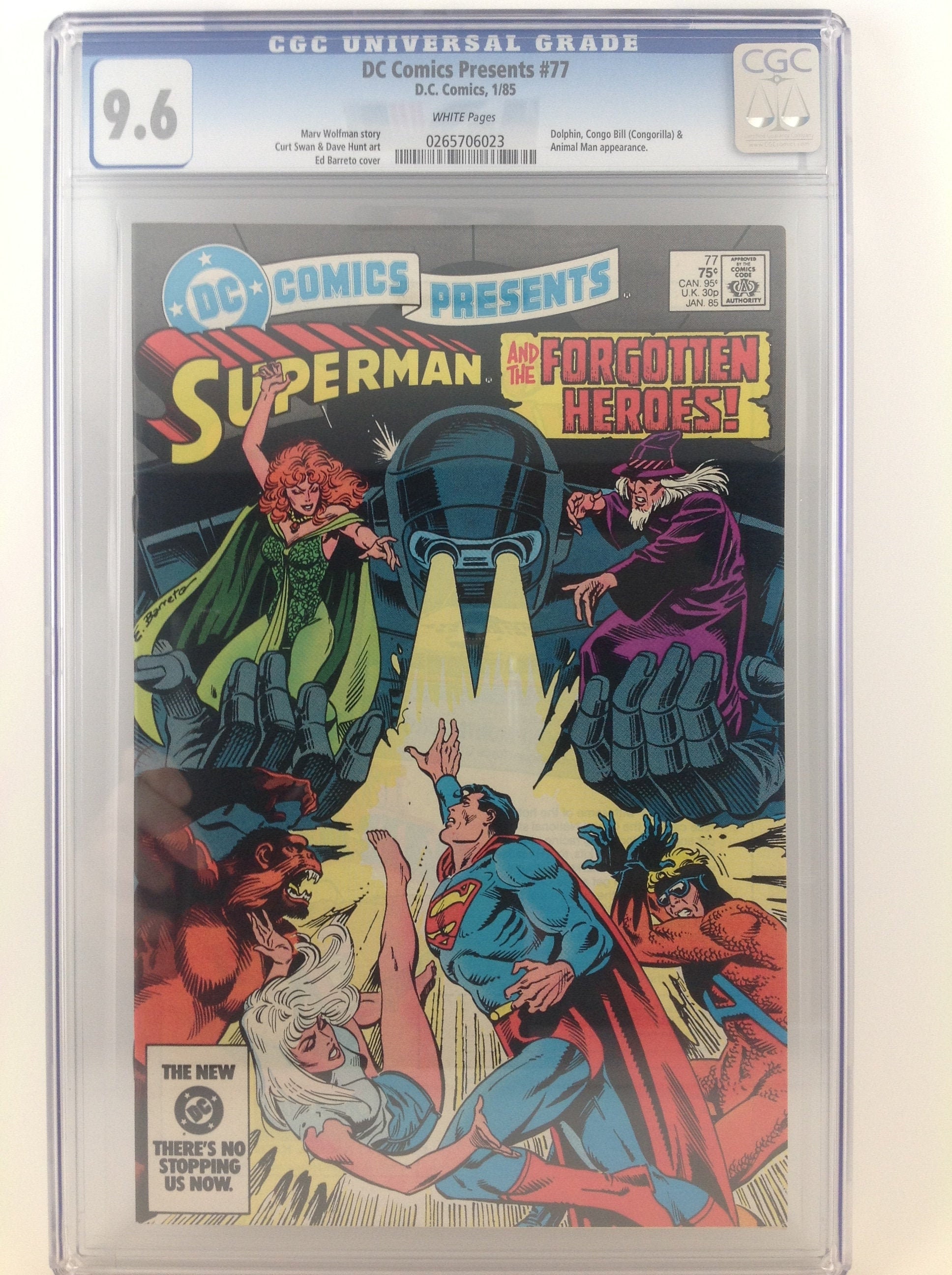Displayed in a pristine CGC universal grade plastic case with a top rating of 9.6, this collectible DC comic book titled "DC Comics Presents Superman and the Forgotten Heroes" showcases vibrant and nostalgic artwork. At the top of the comic, blue and red 3D lettering spells out "Superman" alongside "and the Forgotten Heroes." The scene is vividly colorful, featuring hues of purple, yellow, blue, red, and white. Dominating the cover, Superman is centrally positioned, receiving a shower of light while flying up to face an array of figures. These include a formidable robotic antagonist with outstretched arms and yellow gleaming eyes, a woman dressed in green who points assertively, and a wizard-like character in a purple robe and hat. The background reveals additional characters and a hero line-up across the bottom, reinforcing the classic, action-packed comic aesthetic. This highly graded and well-preserved issue is emblematic of an era when comic books captivated the imaginations of children everywhere.